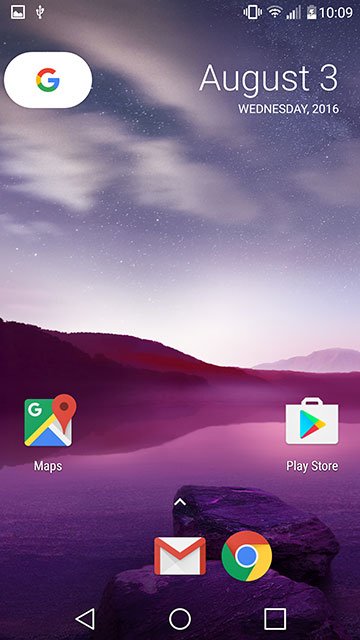This image is a screenshot taken from an Android smartphone running the Lollipop version of the operating system. The indication is based on the design of the navigation bar at the bottom and the user interface style at the top. 

At the top of the screenshot, the status bar features several icons. On the top left, there's a square emblem for the gallery, suggesting that a picture has been taken. Next to it, a USB symbol indicates that the phone is connected via USB. Moving to the right side of the status bar, a vibrate symbol shows that the phone is set to vibration mode. 

Additionally, a Wi-Fi icon displays a connection strength of four out of five bars. The data connection symbol indicates a medium-strength data connection, about halfway full. The battery icon reveals the battery is at approximately 25% and currently charging, as evidenced by the small lightning bolt. The time displayed is 10:09, without specifying AM or PM. 

Just below the status bar, on the top left, the date reads "August 3rd, Wednesday 2016," indicating when the screenshot was taken. On the top right, there's a distinctive "G" emblem encircling white text, signifying a Google search bar.